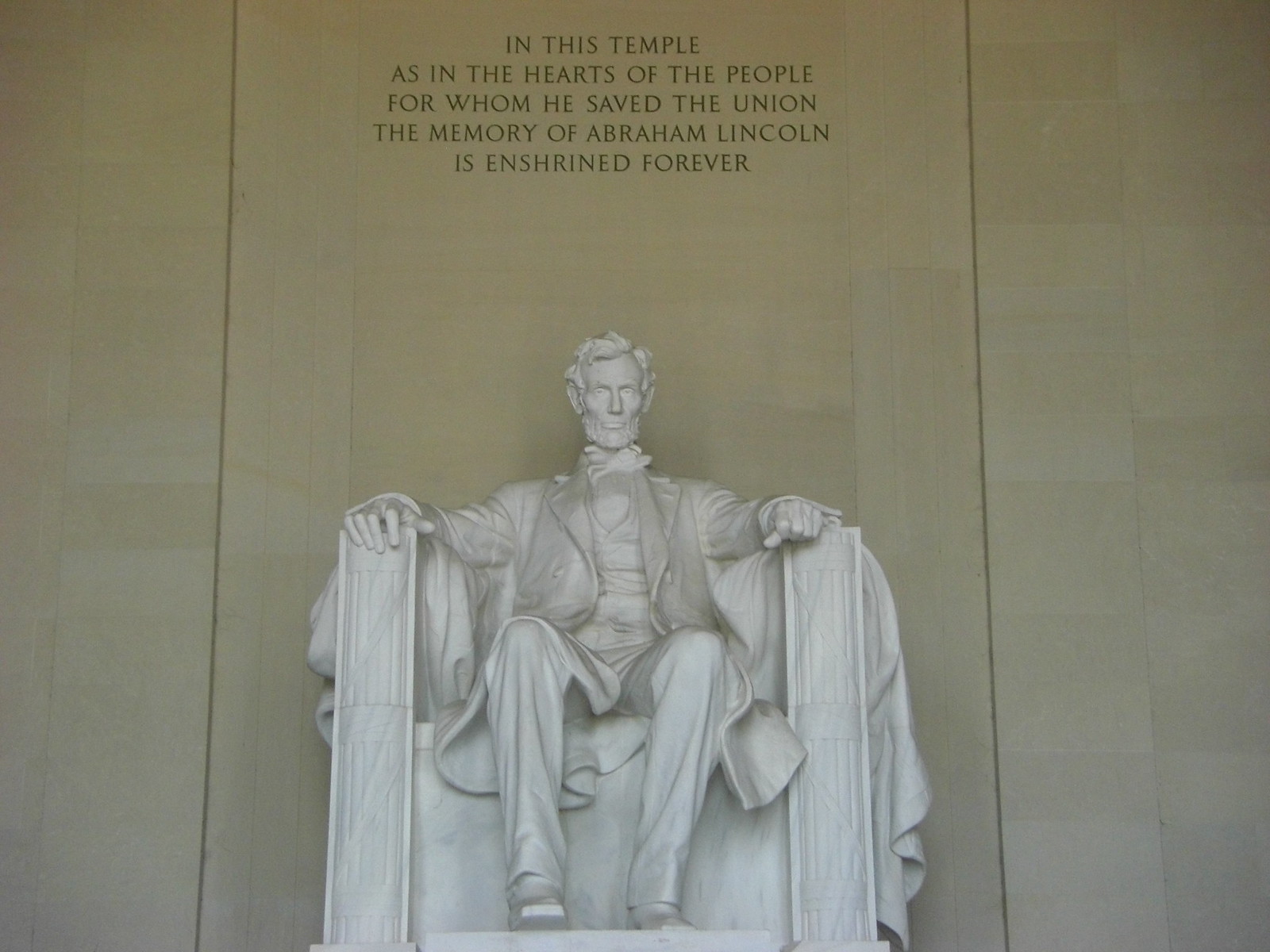This image showcases the iconic white statue of Abraham Lincoln sitting confidently in a large chair, reminiscent of a throne, with his hands resting on the armrests. Lincoln is adorned in a suit with long pants and a bow tie, exuding a sense of solemn dignity. The statue is set against a prominent grey-beige wall that bears a poignant inscription in dark grey or black letters: "In this temple, as in the hearts of the people for whom he saved the Union, the memory of Abraham Lincoln is enshrined forever." This profound tribute encapsulates Lincoln's enduring legacy. The setting, likely to be the Lincoln Memorial in Washington, D.C., adds to the majesty and historical significance of the statue. Shadows cast on the statue create depth, highlighting its detailed craftsmanship.